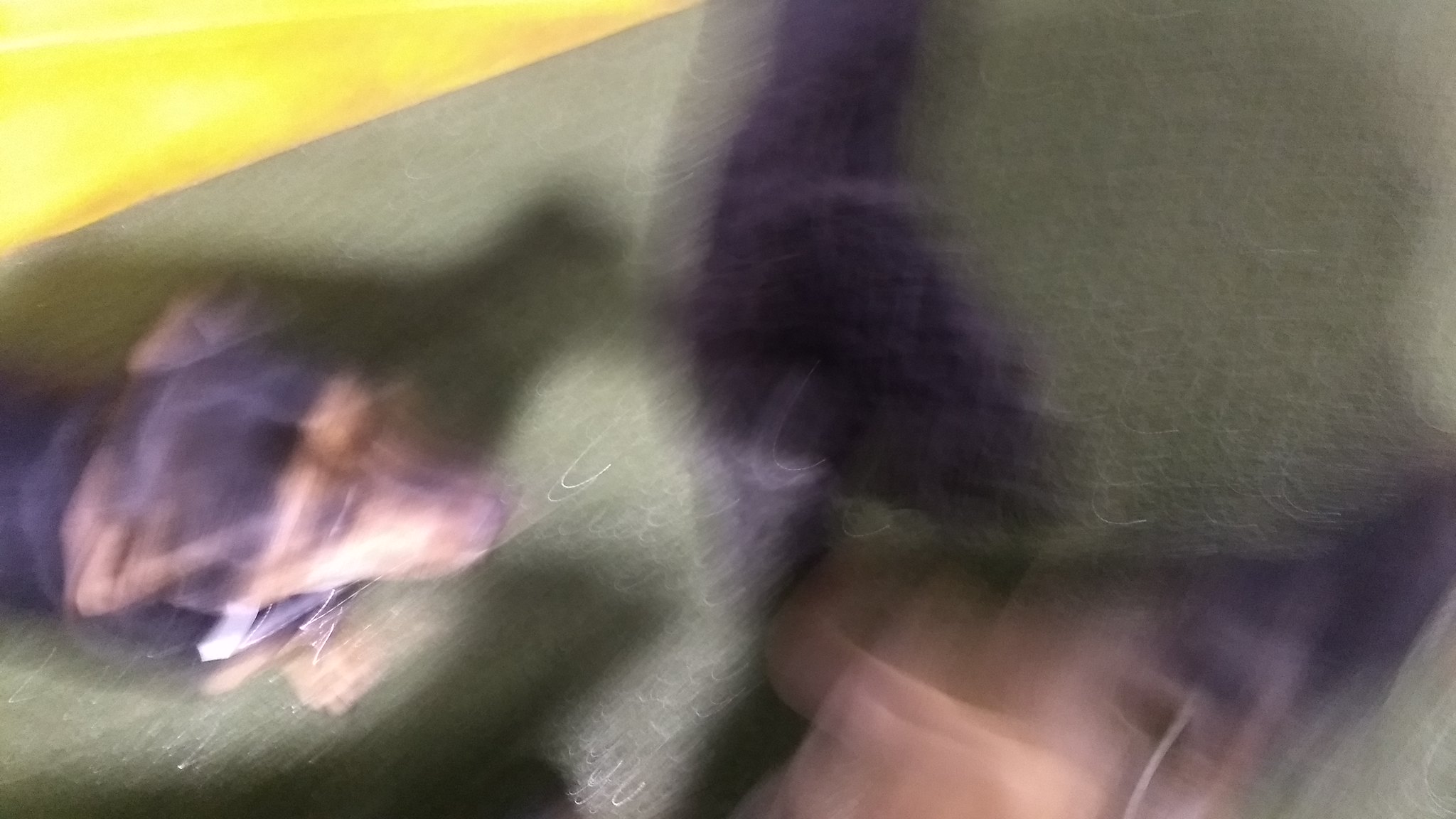In this blurred photograph, the upper left-hand corner features a distinct and bright yellow triangular shape. Below this, there is what appears to be a green couch. Sitting on the couch is a small dog, identifiable by its light brown pointy nose. The dog has black fur on top with light brown ears, although the rest of its body is not clearly visible due to the blurriness. To the right of the dog, there is a continuation of the green blur, likely part of the same couch. In the lower right-hand corner, there is a fleshy-colored shape that seems to be a person's profile, possibly lying down.